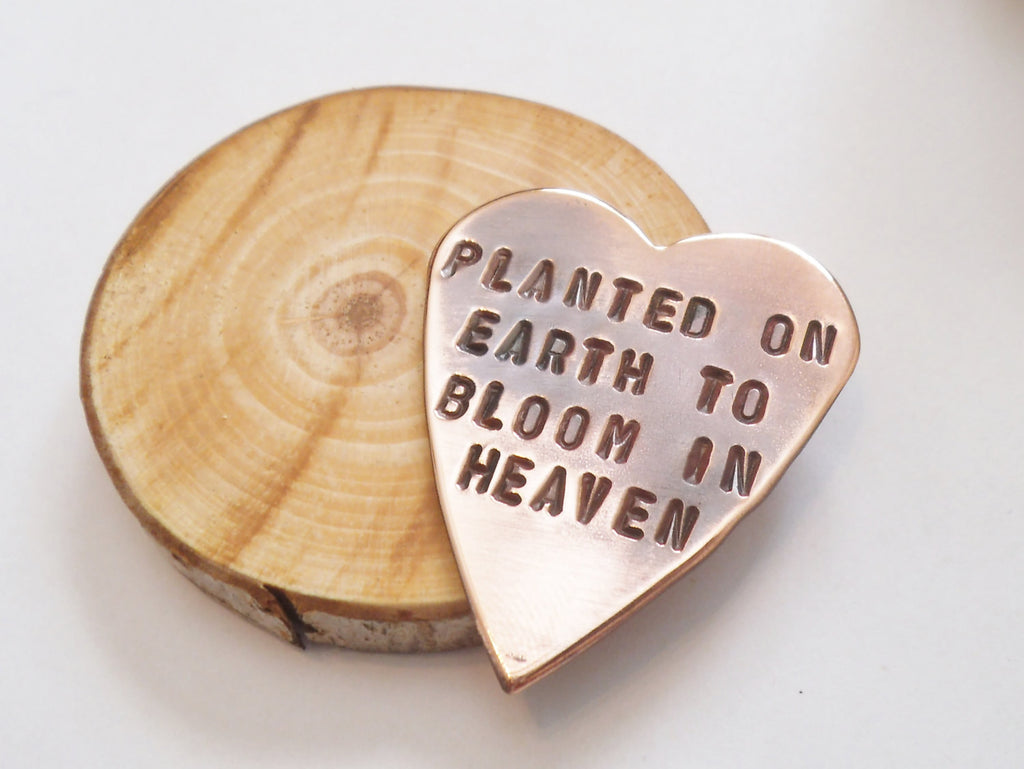The image depicts a close-up photograph of a circular slab of wood, cut from an actual tree trunk, retaining its natural bark around the edges. The bark is whitish-brown, providing a rustic contrast to the smoother, sanded surface of the wood. You can clearly see the age rings and some subtle marks left by a chainsaw across the light brown interior. Resting slightly to the right side of this miniature log slice, roughly the size of a human thumb, is a heart-shaped medallion made of a material resembling copper. The metal heart bears an engraving that reads, "Planted on earth to bloom in heaven." The scene is set against a simple white background, enhancing the natural and artisanal elements of the wood and the engraved pendant, which is artfully displayed on the wooden surface.